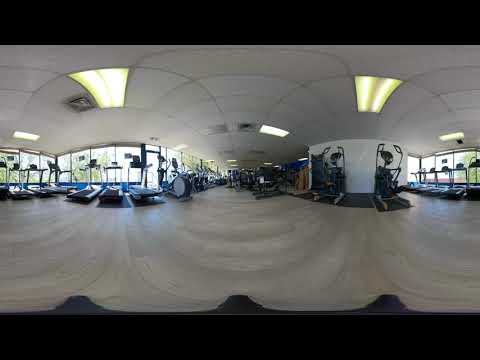The image depicts the interior of a spacious, sophisticated gymnasium characterized by its domed ceiling with skylights and numerous ceiling lights illuminating the space. The gym is predominantly white, with a light gray floor and black or dark-colored exercise equipment. Surrounding the perimeter of the gym, large windows allow natural light to flood in, offering views outside. Numerous treadmills line both the left and right sides of the gym, positioned to face the windows. The central area is filled with a variety of other exercise machines, including elliptical bikes and weight equipment, extending towards the background. In the right foreground, there is a small white cubicle with unidentified objects leaning against it, likely more exercise equipment. The photo appears to be taken from a considerable distance, capturing the extensive layout and sophisticated nature of the gym.